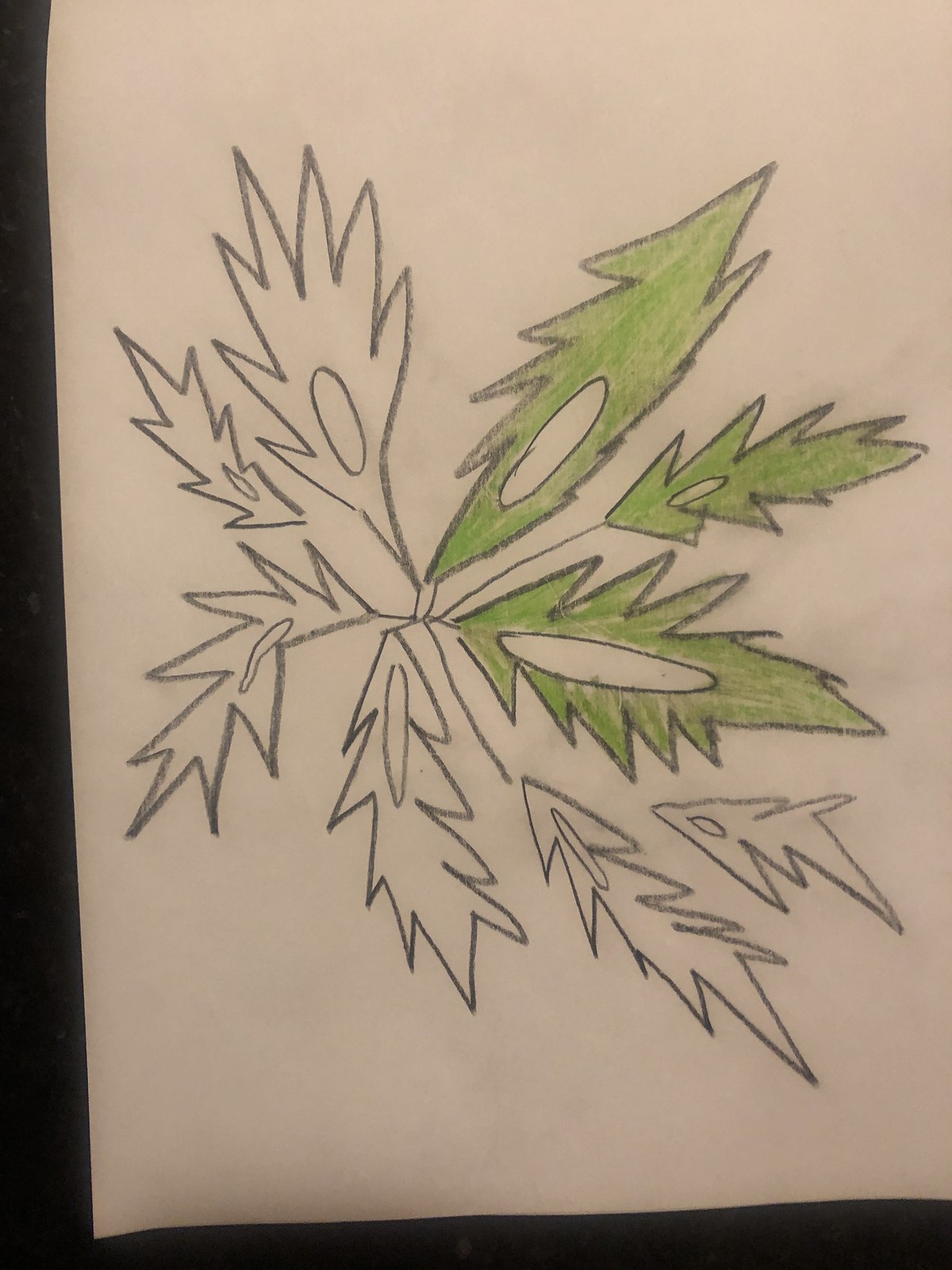Set against a solid black background, an off-white, almost tan, piece of paper displays a captivating design drawn in pencil, possibly charcoal. The main motif consists of a series of zigzagging, pointy lines resembling leaves or shuriken, the traditional Japanese stars. Each of these intricate forms features a central hole, enhancing their resemblance to shuriken. Notably, three forms located on the top right half of the image are filled with a medium-tone green, adding a splash of color to the predominantly monochrome artwork.

The entire composition radiates from a central point, with the zigzagging motifs emanating outward in an arrangement that loosely mimics the positioning of clock numbers. On the right side of the paper, several designs span from the 1 to the 5 o'clock positions. There's an additional form at the 6 o'clock position, and then the imagery continues on the left side at the 8, 10, and 11 o'clock positions. This inventive layout and the convergence of natural and geometric shapes create a dynamic and visually stimulating piece.